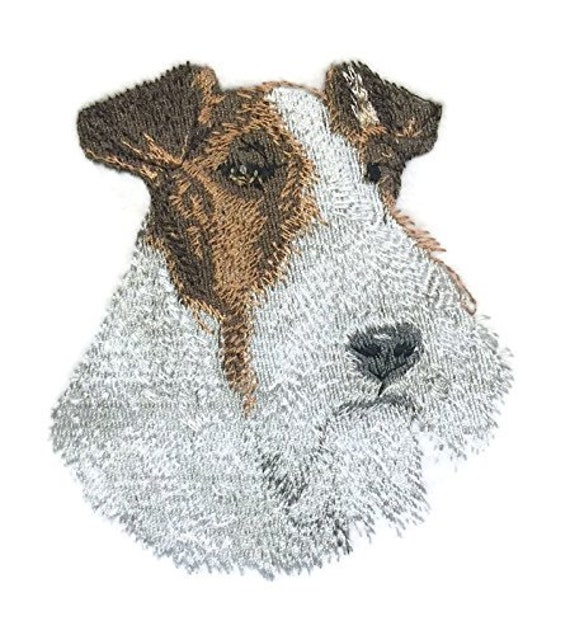A handmade textile piece depicting a dog appears to be either a rug or a detailed sketch mirroring a knitting style. The majority of the dog's face and neck are rendered in white, while brown fur highlights the areas around both eyes. The craftsmanship suggests a completed work with a smooth texture, although it may not have the precision of a professional creation. Despite some roughness, the distinct sections of the dog's face and different fur colors are clearly recognizable. The overall appearance leans towards a rug-like form, though its exact classification remains uncertain.